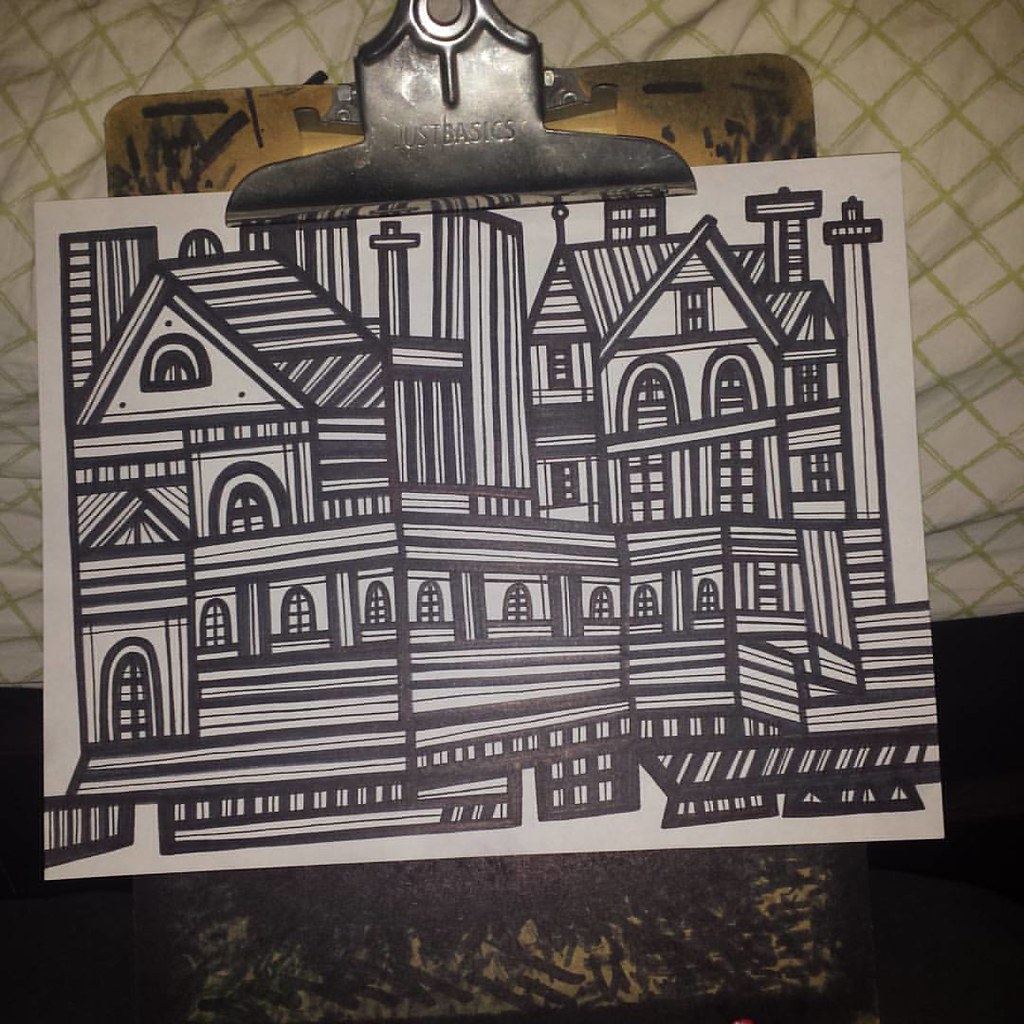An artist's sketch, rendered in black marker on a clean white sheet of paper, is securely attached to an aged clipboard bearing the brand name "Just Basics" on its metal clip. The wooden clipboard surface is adorned with various black marker scribbles, adding to its well-used character. The sketch itself portrays a dynamic downtown scene, featuring a series of townhouses and taller structures, some crowned with spires. The intricacy extends to a sidewalk, bringing the bustling urban landscape to life.